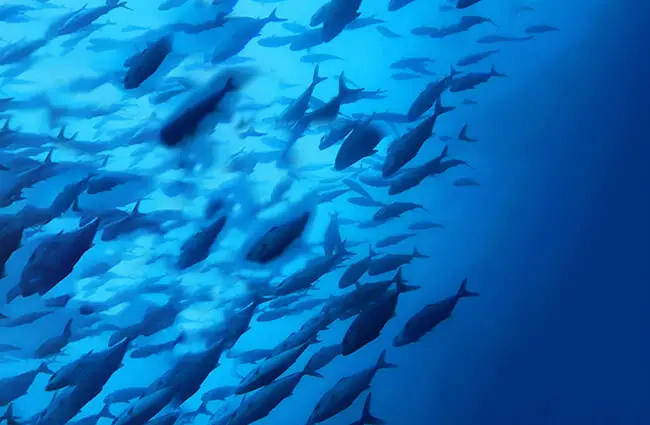This underwater landscape photograph features a mesmerizing school of small fish swimming from the upper right corner towards the lower left corner. The scene is dominated by shades of blue, transitioning from a deep, dark hue to a lighter, glowing tone on the left. The image provides a unique vantage point, looking up towards the water's surface, possibly with sunlight reflecting. The fish, shown in various levels of clarity, form a diagonal pattern, emphasizing their collective movement. While the right side of the image offers a clearer view of the blue water, the left is densely populated with the silhouettes of hundreds of fish, showcasing their synchronized motion and varying proximities.